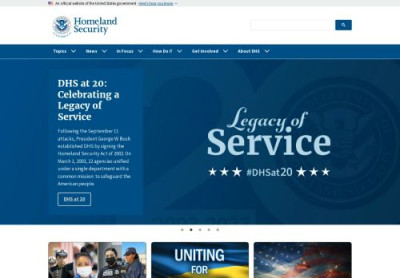The image is a horizontally oriented web page, likely from a website accessible via desktop, laptop, or smart device. 

At the top of the page, there is a long gray strip featuring an American flag followed by black text and blue underlined text, though the specifics are blurred. Below this is a white background, standard for many computer screens. On the left side, the Department of Homeland Security (DHS) logo is prominently displayed, accompanied by the text "Homeland Security" in blue lettering. 

On the far right of the page, there is a white search bar with a blue magnifying glass icon for initiating searches. 

The main content area features varying shades of blue as the background: navy, dark, and medium blue hues. There are white, clickable elements at the top for additional information. The central text reads "DHS at 20: Celebrating a Legacy of Service," with a brief blurb underneath. The phrase "Legacy of Service" is flanked by three stars on either side, followed by the hashtag "#DHSat20" and another row of three stars.

Below this text are several gray circles, indicating the presence of multiple images that users can scroll through. At the bottom, three images are displayed, possibly related to the legacy of service theme.